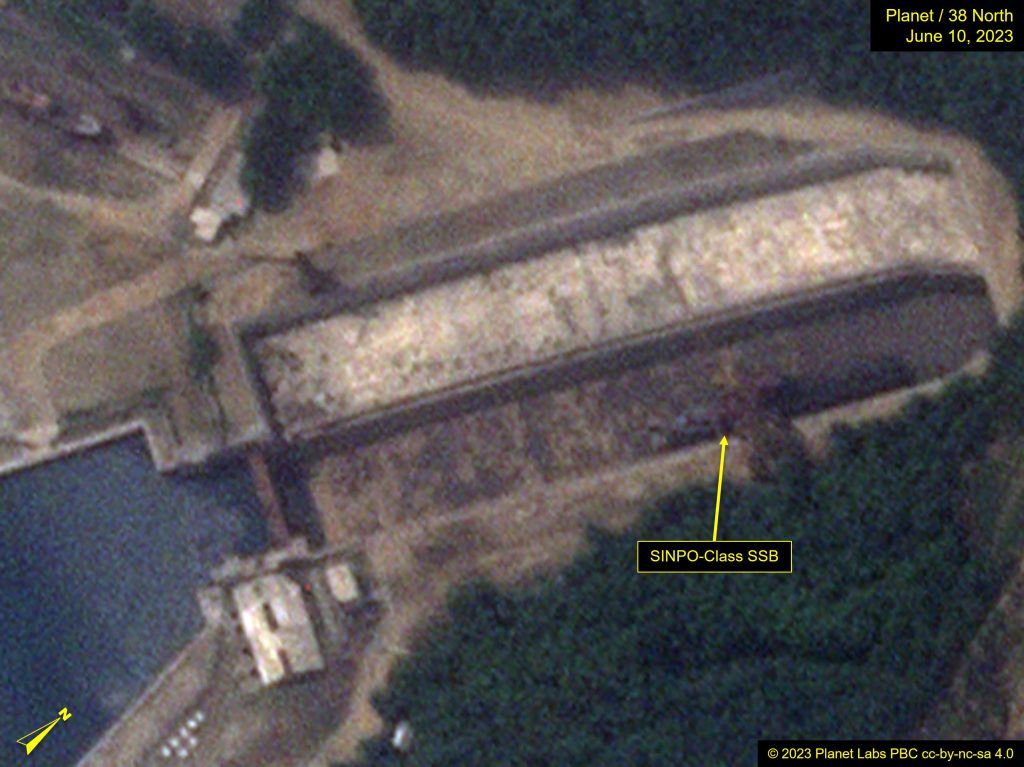This detailed satellite image captures an aerial view of a location with a specific area marked by a prominent black label with yellow letters stating "SINPO-class SSB." A yellow arrow emanates from the label, pointing towards a blurry object in the center of the image, making it challenging to identify. Surrounding this labeled object, there's a notable density of trees below, to the right, and above it, while a small body of water is visible to its left. The photograph also includes a portion of a compass indicating north. In the bottom right corner, there's a "Copyright 2023 Planet Labs PBC CCBY NCSA 4.0" notice, while the top right corner reads "Planet / 38 North June 10th, 2023." The image appears to depict areas of greenery, grass, and some cleared land possibly indicating constructed structures or removed vegetation, along with a suggestion of boats in the water area, despite the overall blurriness of the photograph.